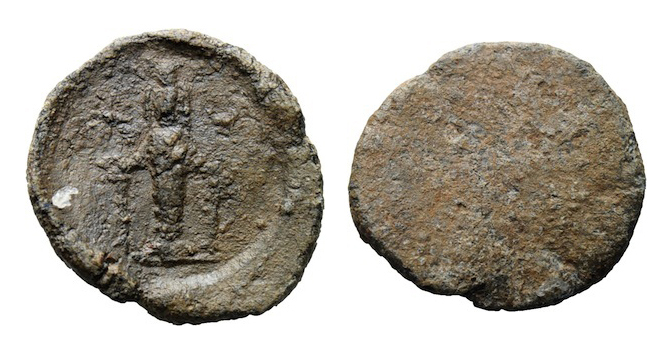This image showcases the front and back of an ancient coin, possibly Greek or Roman. The coin, predominantly dark gray with patches of brown and green, is carved from a material that seems to be a blend of metal and stone. Its overall shape is roughly circular but displays irregularities, such as chips and an arching protrusion on the lower bottom right, adding to its ancient and worn appearance.

The front side of the coin features a prominent figure etched in the center, resembling a person standing on a pedestal. This figure appears to be interacting with another figure that has extended arms and a missing head, framed by vertical bars. The intricacies of the scene are challenging to discern due to the coin's age and wear.

On the reverse side, the coin is markedly pitted and lacks any discernible imagery. Instead, it is characterized by a blend of flat, rocky textures in hues of brown and light green, further emphasizing its ancient origins. The background of the image is white, which starkly contrasts with the dark, earthy colors of the coin, highlighting its detailed etchings and time-worn features.